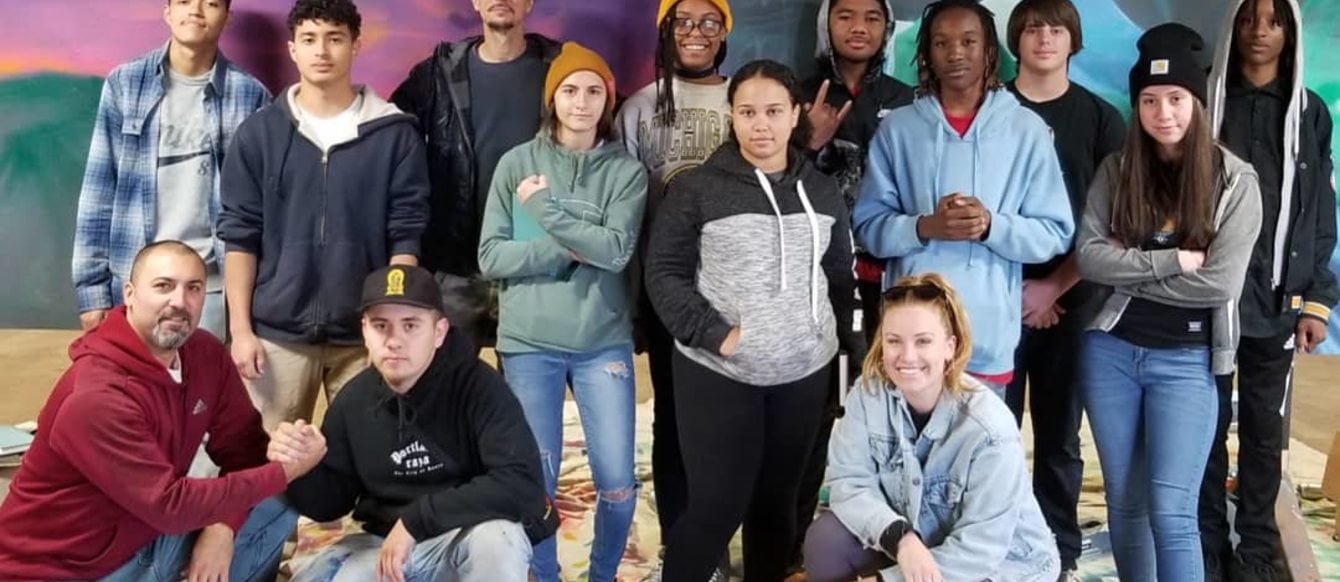The image depicts a vibrant group of possibly 14 people, potentially students, gathered together, likely for a class or club photo. The setting suggests an artistic environment, indicated by the painted wall in the background featuring hues of purple, blue, green, and yellow, with a canvas strewn on the floor behind them. In the front row, two individuals are crouching; on the far left, a man in a red hooded sweatshirt, who appears to be older and may be a teacher or coach, kneels next to a person in a black cap and shirt. The detailed attire of the group shows a blend of casual outfits: people are dressed in hooded sweatshirts, jeans, track pants, t-shirts, and some don baseball or wool hats.

In the back two rows, starting from the left, there is a person in a blue-colored plaid shirt with a white undershirt bearing a black Nike Swoosh, next to them is someone in a blue hoodie matched with cream-colored pants. Further right, a woman in an orange hat, gray shirt, and blue jeans stands alongside another in a yellow hat, glasses, and a gray "Michigan" shirt paired with dark pants. A person rocks a gray hooded sweatshirt with a black hooded shirt underneath, signaling with a rock and roll hand gesture. Another woman stands in a gray and black colored hoodie with black sweatpants, adjacent to someone in a light blue hoodie revealing a red shirt underneath. The crouching woman in front is attired in a whitish jean jacket with dark pants, while behind her stands a person dressed entirely in black. Next, a man in a gray hoodie with black accents wears all black further to the right, standing beside a woman in a black hat, black shirt, gray hoodie, and blue jeans.

Each individual’s unique attire and positions create a lively and diverse scene, captured against a creatively colorful backdrop, possibly representing an art class or creative project group.